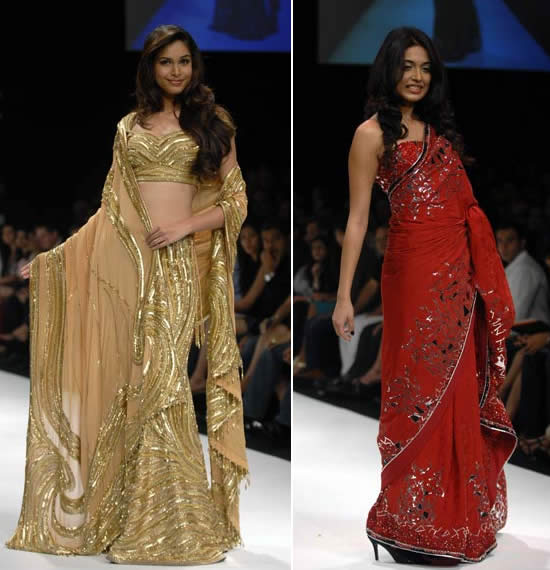This image features a side-by-side composition of two models on a white catwalk, set against a backdrop of spectators. Both models showcase exquisite saris from Satya Paul, each with long, dark, over-shoulder hair styled elegantly.

On the left, the model stands confidently in a two-piece golden ensemble that includes a midriff-revealing top and a long, flowing skirt. The intricate designs on her outfit add to its sophistication, creating a shimmering effect as she smirks at the camera. Over her shoulders drapes a golden fabric that complements her skirt's form-fitting elegance, and her wavy brown hair cascades over her shoulder, adding to her poised appearance.

On the right, the model is adorned in a striking red sari embellished with sparkles and detailed designs. The dress flows gracefully to the floor with her foot peeking out, revealing a black heel. Her dark, curly hair enhances her sophisticated look as she smiles warmly. Her sari features intricate black and silver patterns that draw the eye, enhancing the dress's overall allure.

Both women are poised on the runway, capturing the essence of high fashion in their elegant, floor-length saris, with the audience's gaze fixed upon them in admiration.